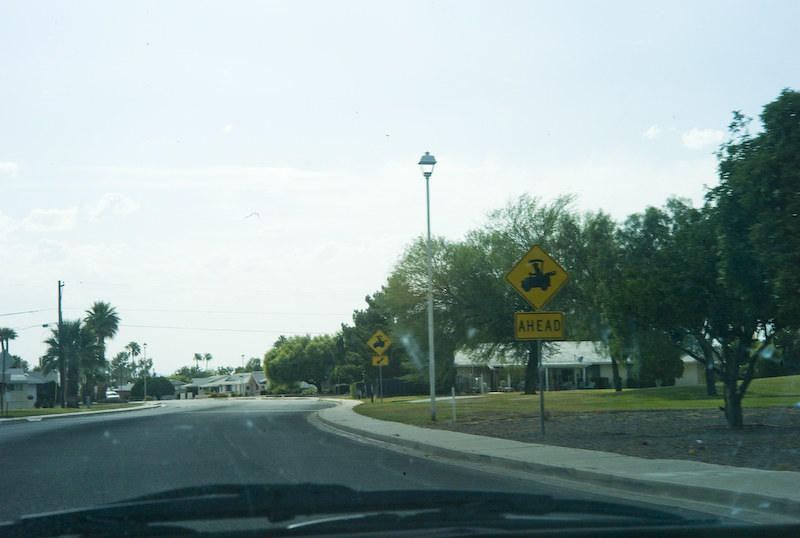A daytime photograph taken from the interior of a car driving down a clear two-lane road, displaying bright sunlight and noticeable glare. The windshield, visibly dirty with numerous white streaks and spots, indicates frequent use. On the roadside, there are multiple signs featuring images of tractors accompanied by text warning of tractors ahead. These signs suggest that the area is likely rural or agricultural. The photo captures an ordinary moment in a driver's journey, highlighting the simplicity and tranquility of countryside travel.